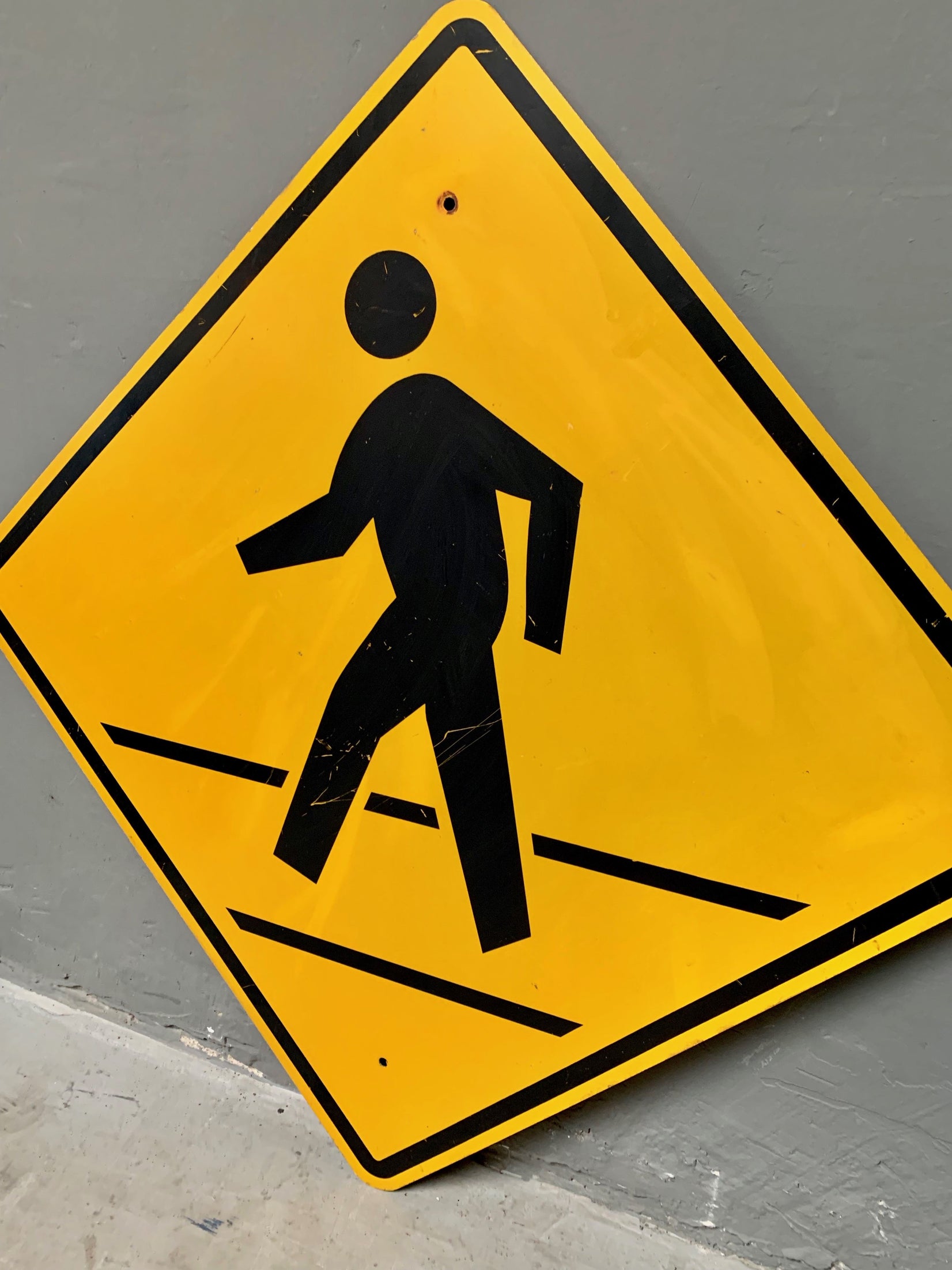The photograph features a yellow diamond-shaped pedestrian crosswalk sign, set against a recently painted gray cement wall with a lighter gray industrial floor. The sign, outlined in black, is tilted at a 45-degree angle. In the center, it displays a black silhouette of a person walking toward the left, characterized by a floating black head and two parallel lines beneath, suggesting a road. The silhouette also has a notable single black spot. The sign shows signs of previous mounting, with two unused screw holes, indicating it was either recently removed from a pole or is awaiting installation.